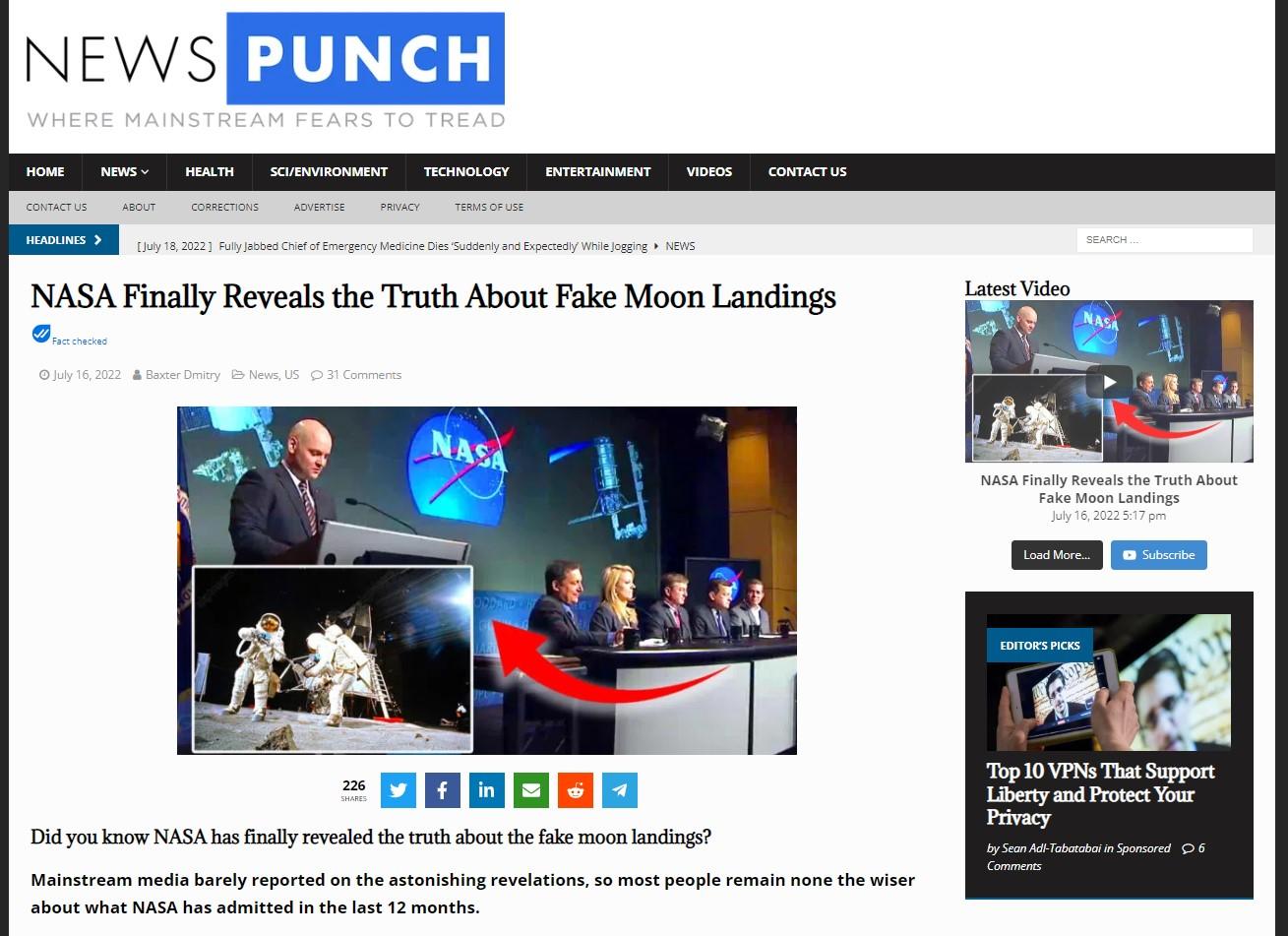The screenshot features the homepage layout of a website named "News Punch." The structure is outlined with black stripes framing the left, bottom, top left to bottom left, top right to bottom right sections. At the top, there is a white background featuring the "News Punch" logo; the word "Punch" is distinctly set against a blue background. Beneath the logo, the site's tagline, "where mainstream fears to tread," is prominently displayed.

Following the header, there is a black navigation bar with various menu options: Home, News, Health, Sci/Environment, Technology, Entertainment, Videos, and Contact Us. Directly under this, a gray stripe provides additional links: Contact Us, About, Corrections, Advertise, Privacy, and Terms of Use.

The content section of the page continues with a white background. On the upper left, just below the secondary navigation, there is a green button labeled "Headlines" with an accompanying forward arrow. The date mentioned is July 18, 2022. The main headline reads: "Fully jabbed chief of emergency medicine dies suddenly and unexpectedly while jogging," indicating the website’s leaning towards conservative and potentially controversial topics.

Directly beneath this is another headline: "NASA finally reveals the truth about fake moon landing," accompanied by an image of a NASA press conference, which implies the propagation of conspiracy theories. The exaggerated presentation and selection of news hint at the website's inclination towards sensational and possibly fabricated news stories.